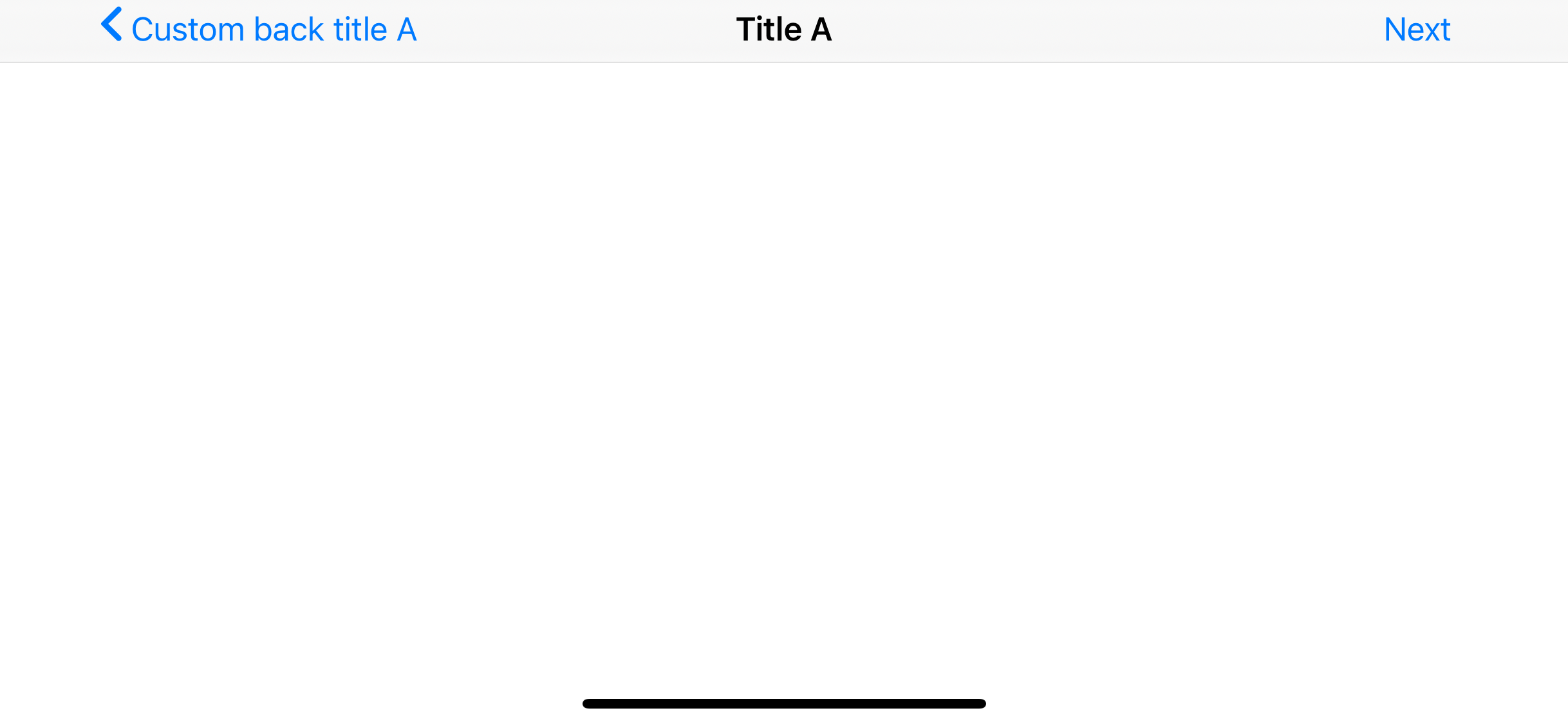The image predominantly features a stark, blank background with a light gray rectangle positioned on the left side. Within this rectangle, there is a blue arrow pointing towards the left. Accompanying the arrow, the text "CUSTOM BACK TITLE" is presented in uppercase, with each letter of "CUSTOM" (C-U-S-T-O-M), "BACK" (B-A-C-K), and "TITLE" (T-I-T-L-E) depicted in a bold, blue font.

Centered within the image, there is a bold, black text that reads "TITLE A," with each letter including the "A" capitalized (T-I-T-L-E A).

On the right side of the image, the text "NEXT" appears in a non-bold, blue font (N-E-X-T), creating a contrast with the previous black bold text.

Towards the bottom of the image, there is a small, dark navy blue oval that resembles a scrollbar extending across the lower edge. The overall layout leaves considerable white space, offering a minimalist design.